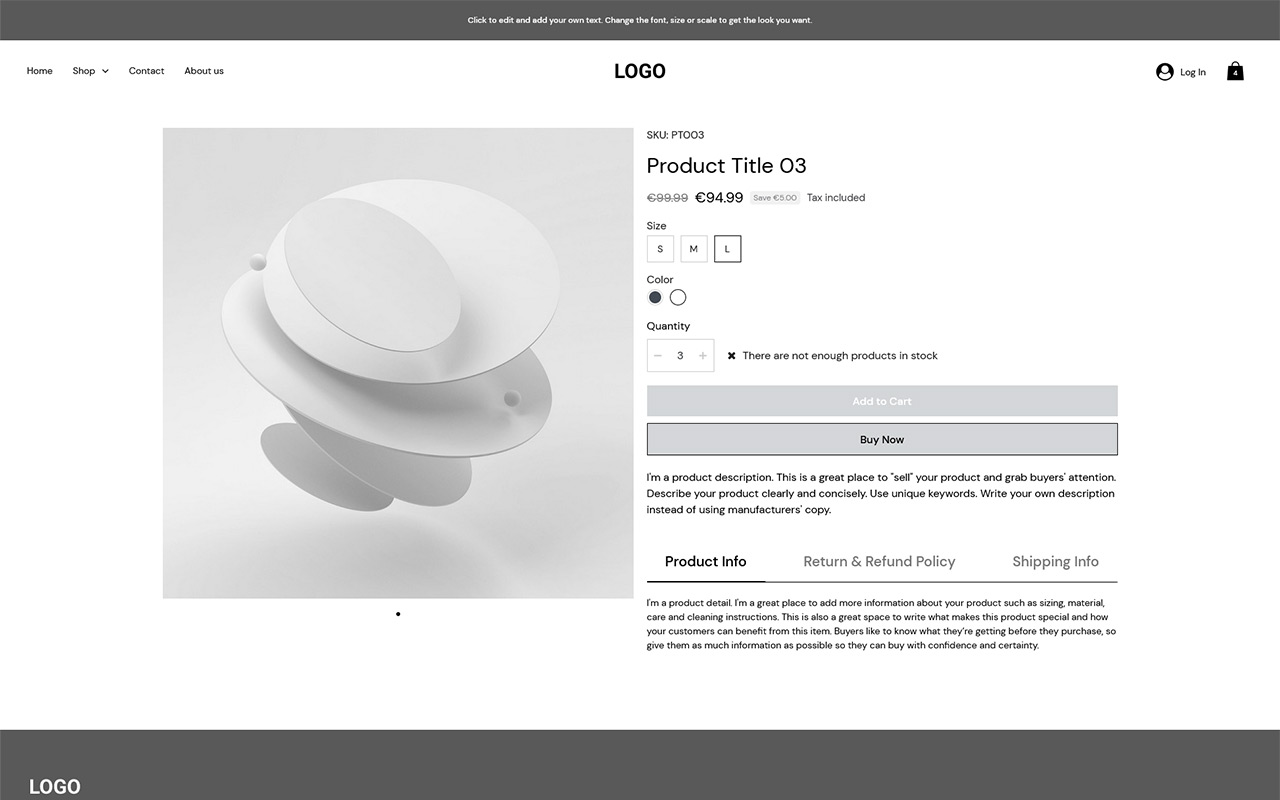This image is a screenshot of a web page with a greyscale color scheme consisting of grey accents on a predominantly white background. The layout is framed by grey blocks both at the top and bottom of the screenshot.

The web page is a template design, intended for users building a website, specifically showcasing a product layout. The template features distinct sections for various product details, allowing customization by replacing placeholder text with actual product information.

Currently, the placeholders include:
- **Product Title:** "Product Title 03"
- **Product Description:** "I'm a product description"
- **Product Info Section:** "I'm a product detail"

These placeholders serve as guides for users to input their own specific information, providing a clear structure for product presentation on the finalized website.